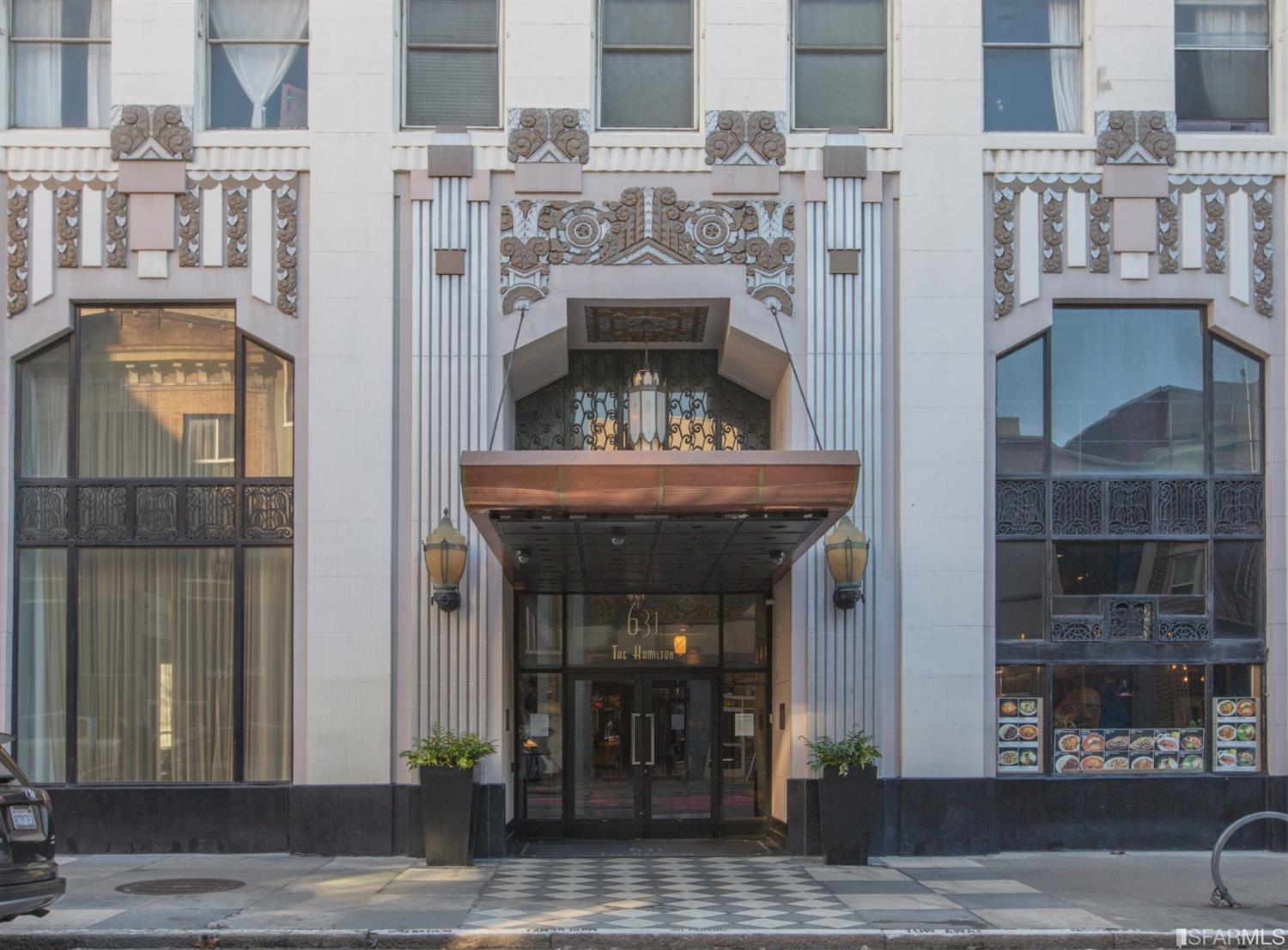This photograph depicts the exterior of a modern, tall, and wide building showcasing Art Deco architecture. The structure is primarily composed of white and beige concrete, featuring highly intricate elements. At the center of the image, a prominent double glass door forms the entrance, adorned with a golden inscription reading "631 the Hamilton." 

Above the entrance is a black and brown awning, extending from the roof. Flanking the entryway, two sizable black planters, containing vibrant green plants, are positioned on either side. Complementing these features, old-school lamps in black and amber hues are mounted above the planters on the wall.

The sidewalk leading up to the entrance displays a gray and beige checkerboard pattern. Two large windows, one on the left and one on the right, bookend the ground floor, with the window on the right revealing images of food, suggesting an adjacent restaurant. The second floor includes a row of windows, hinting at potential hotel rooms above. 

Overall, the combination of Art Deco details, modern materials, and the inviting entryway emphasizes the elegance and historical essence of 631 the Hamilton.